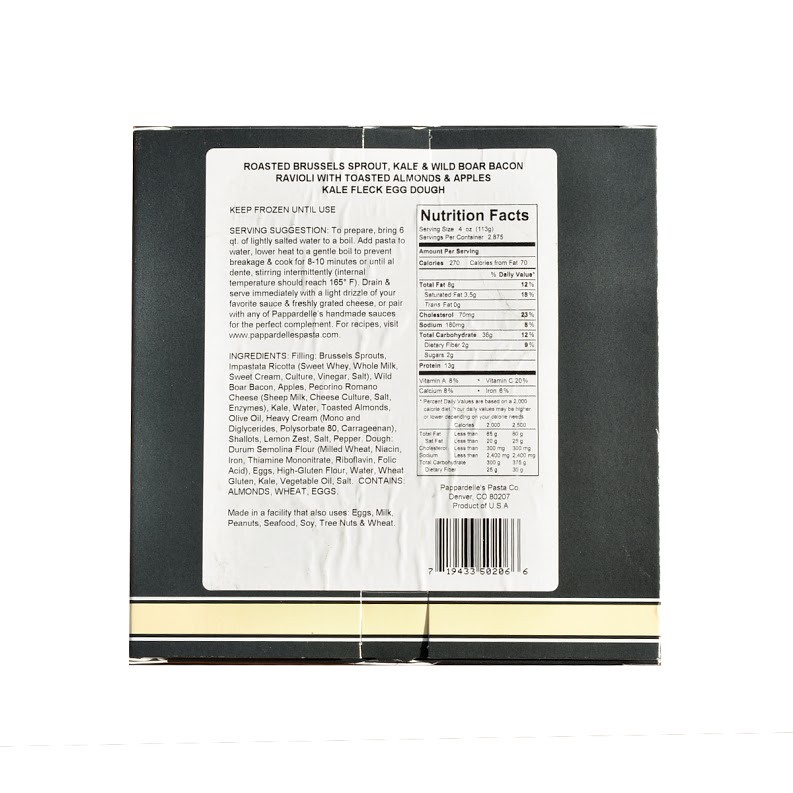This image is a nearly square, high-resolution photograph, almost resembling a scan, of a label on the back of a black food box. The box features a distinctive thin yellow bar at the bottom, flanked by thinner white bars above and below it. Dominating the image is a large white label that details the contents and characteristics of a pre-packaged frozen meal. The meal is identified as roasted Brussels sprout, kale, and wild boar bacon ravioli with toasted almonds and apples, encased in kale-flecked egg dough. The primary right side of the label showcases a standard nutrition facts panel, listing calorie count (270 calories per serving), total fat, cholesterol, sodium, total carbohydrates, and protein content, among other nutritional values. On the left side, the label provides the ingredients, serving suggestions, and instructions to keep the item frozen until ready to use. The bottom right corner of the label features a barcode, completing the typical elements found on food packaging.